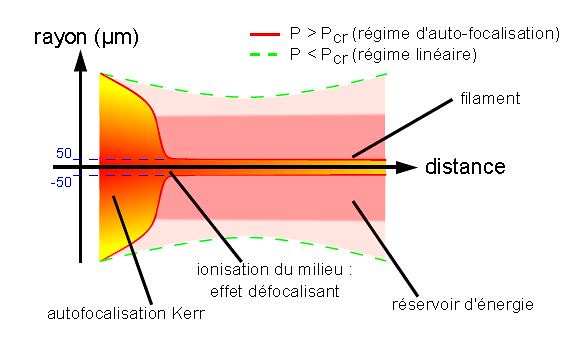This image depicts a detailed scientific diagram, predominantly annotated in French, illustrating various aspects of what appears to be a study on energy dispersion and focal effects in a medium. 

On the left side of the diagram, there is a fiery, semi-circular blob featuring a gradient from intense red at its core to a yellowish hue at the periphery, resembling the appearance of the sun. Extending from this fiery half-circle is a protuberance sharing the same color scheme, symbolizing a filament. An arrow runs through this filament, directing towards the term "distance."

Above this region, another arrow points upward, labeled "rayon," accompanied by a scientific symbol. The background is tinged pink, scattered with green indicator lines that display the dispersion of energy. 

While the rest of the diagram is in French, key terms identified include "autofocalization curve," "ionization du milieu," "effet de focalisation," and "réservoir de l'énergie," suggesting a complex interplay of focus effects, ionization in the medium, and energy storage.